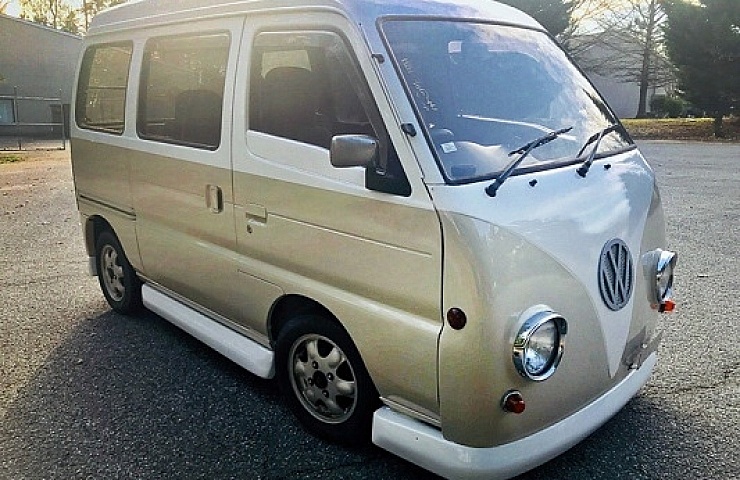In the center of the image is a retro-looking Volkswagen minivan, exuding classic charm. The front of the minivan bears a resemblance to the head of an insect, with circular headlights that look like large eyes and a front bumper that mimics a mouth. The van is painted in a light purple, almost light gray hue, with white accents adorning various parts including the bumper, sides, and roof. Its windshield wipers are visible, adding to the detailed appearance of this seemingly small vehicle.

The minivan is parked in an empty parking lot, with a gray asphalt surface visible beneath it. In the background, large houses can be seen, suggesting a suburban setting. To the right, there is a field of grass with some trees, further enhancing the picturesque scene.